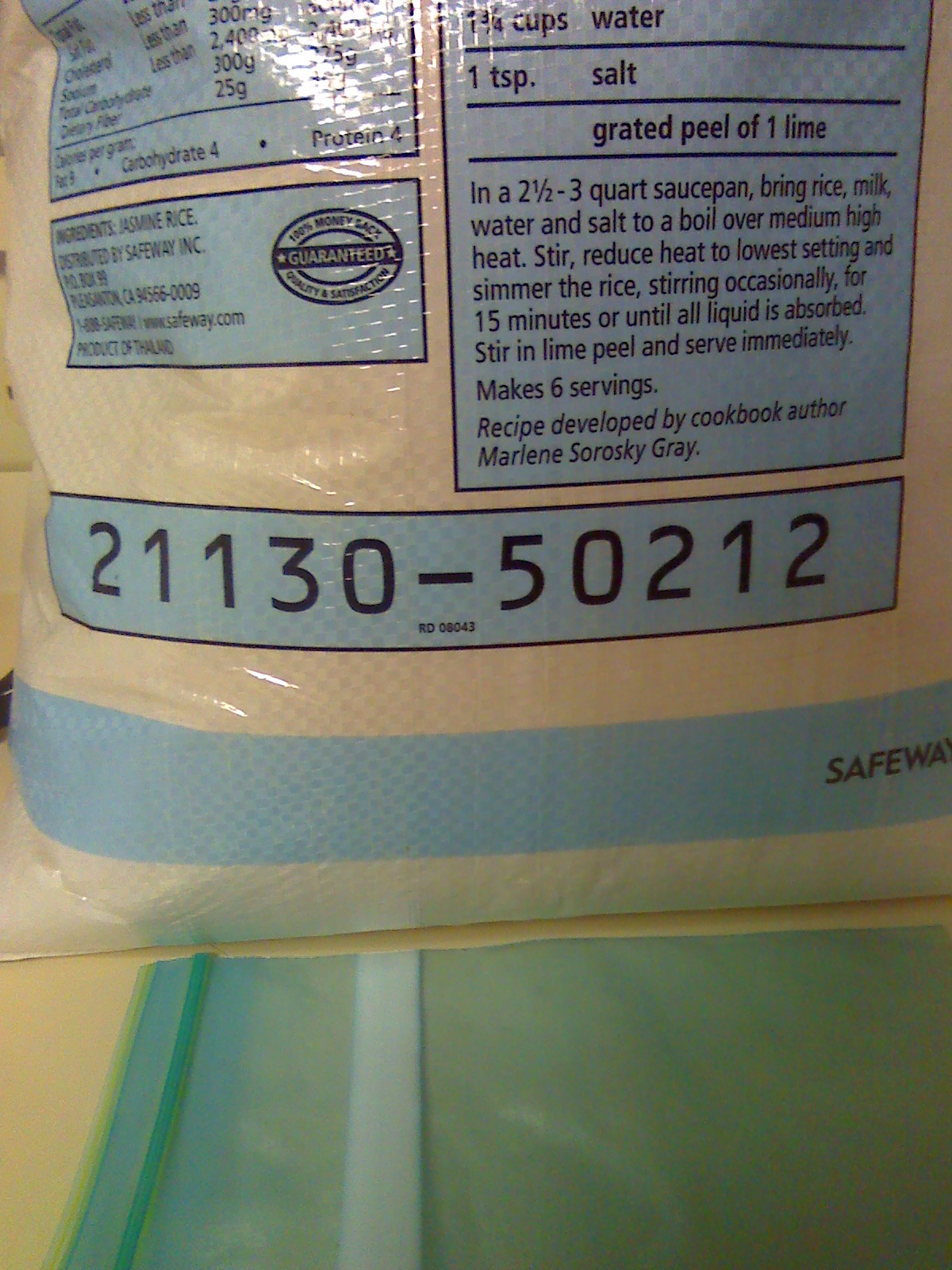This image depicts a plastic grocery store bag containing a package of jasmine rice. The rice bag features a distinctive light blue strip encircling its bottom portion. On the right side of the bag, the word "Safeway" is printed, indicating the store of origin. The top section of the rice bag contains nutritional information, albeit partially obscured as it's cut off about halfway. In the top left corner of the bag, there are two squares—one small and one large—side by side, with the larger square being partially cut off. The packaging also includes cooking instructions, guiding the user to prepare the rice in a two and a half to three quart saucepan with rice, milk, water, and salt. This instruction section is underscored by a bold strip displaying a prominent number.